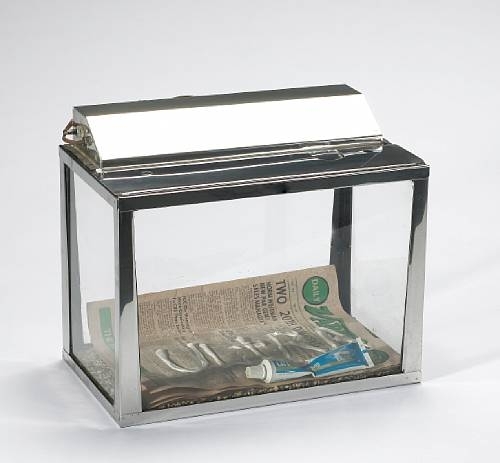The image depicts an abstract art exhibit featuring a vintage rectangular aquarium with silver chrome edges set against a white background. The aquarium has four clear glass walls and is topped with a hood containing a light fixture, potentially an ultraviolet or standard vapor lamp. Inside the aquarium, the base is covered with a variety newspaper, which prominently displays the word "daily" inside a green circle outlined in black. A partially squeezed blue-and-white tube of toothpaste lies on the newspaper, having been used to write the word "ULTRA" in bold, uppercase letters across the newspaper. The scene inside the aquarium is minimalistic yet striking, blending everyday objects with a creative, artistic presentation.